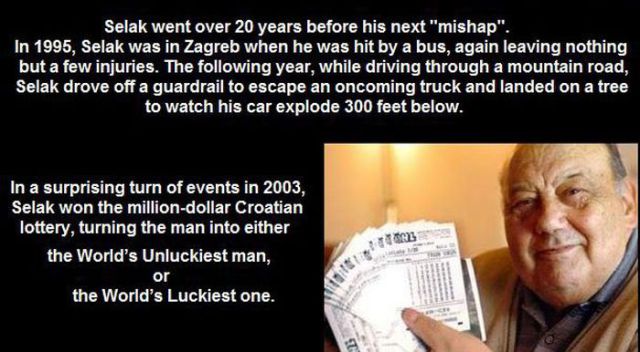The image features a black background with white lettering detailing an extraordinary story of a man named Selick. Highlighted on the right-hand corner is a photograph of an elderly, balding man with short hair, smiling warmly. He wears a sweater vest over a blue button-up shirt and holds a fanned-out stack of lottery tickets. The text recounts Selick's series of astonishing events: In 1995, he was struck by a bus in Zagreb but escaped with only minor injuries. The following year, he veered off a guardrail on a mountain road to avoid an oncoming truck and landed in a tree as his car exploded 300 feet below. The narrative takes a surprising turn in 2003 when Selick won the million-dollar Croatian lottery, sparking a debate whether he is the world's unluckiest man or the luckiest.